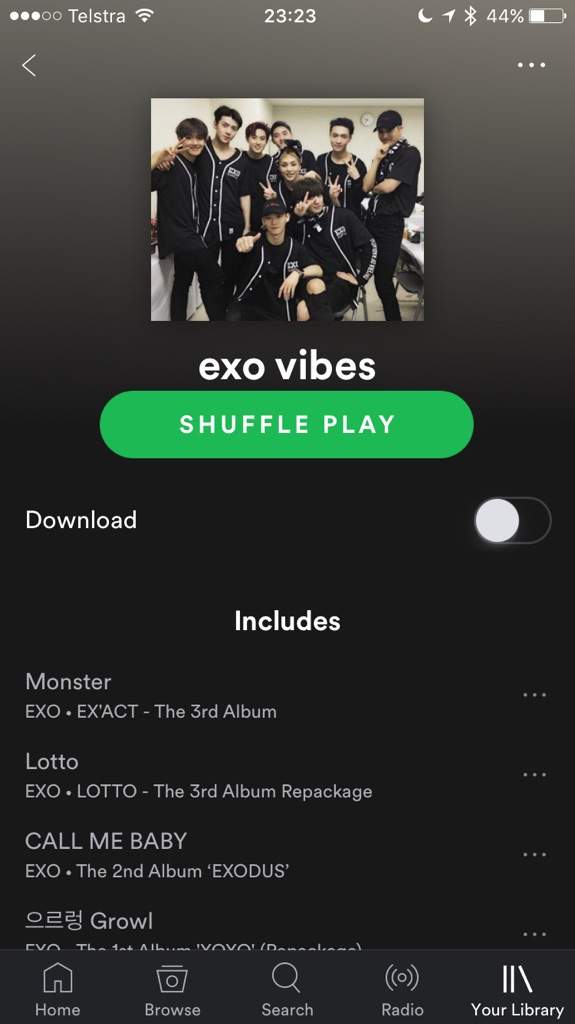Here's a detailed and cleaned-up caption for the described image:

---

The image shows a screenshot of a cell phone display with a battery life at 44%. The device is connected to the internet, with the 'Do Not Disturb' mode active, indicated by a moon icon. The carrier is listed as Testra, and the time displayed is 23:23.

On the screen is an open music streaming application featuring a singing group of Asian artists, all dressed in coordinating black outfits. The group's name, "XO Vibes," is prominently displayed at the top. Below the title, there's a green "Shuffle Play" button on the right and a "Download" button on the left. To the right of the "Shuffle Play" button is an unilluminated, round, white button.

The description includes a list of albums and songs by the group, such as "Monster, XO Exact, the third album," "Lato, XO Lato, the third album repackage," "Call Me Baby, XO, the second album, Exodus," and another title in Asian characters, followed by "Growl."

At the bottom of the phone screen, there are icons and labels for "Home," "Browse," "Search," "Radio," and "Your Library." The overall interface of the app is predominantly black with some gray elements at the top.

---